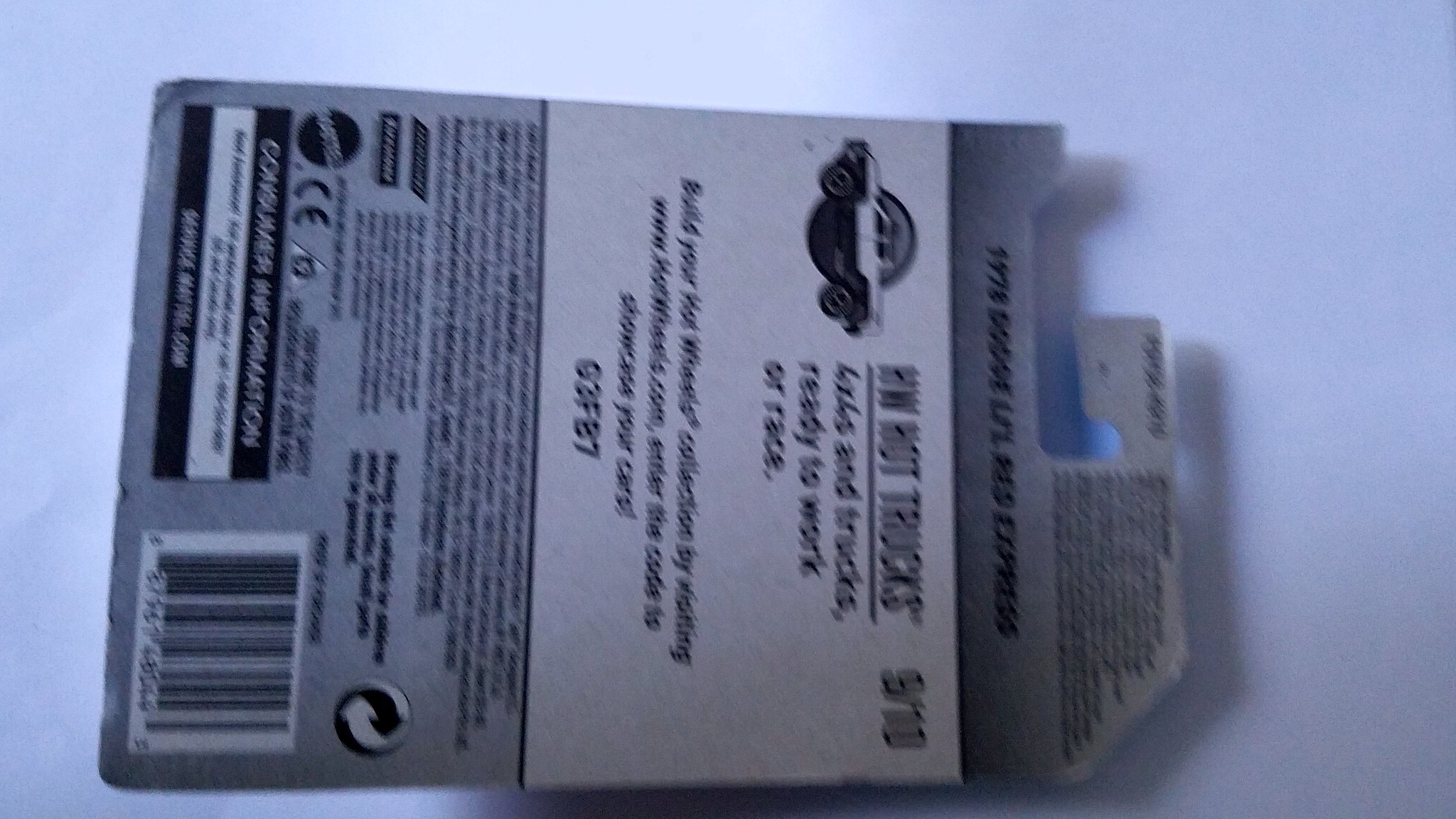This image displays the back of a toy packaging that is somewhat blurry, obscuring many details. The packaging is predominantly black and white and seems to be for a toy car, specifically resembling Hot Wheels products. Notably, it mentions a model, likely a 1978 Dodge truck, under a collection labeled "HW Hot Trucks." The packaging indicates that it is item number 9 out of a series of 10. An illustration of the truck in black and white is present. The description on the packaging suggests the trucks are "ready to work or race" and encourages collectors to "build your Hot Wheels collection." Although much of the text is too blurry to decipher, the packaging appears to be a Mattel Hot Wheels product, confirmed by the visibility of a UPC code on the back.